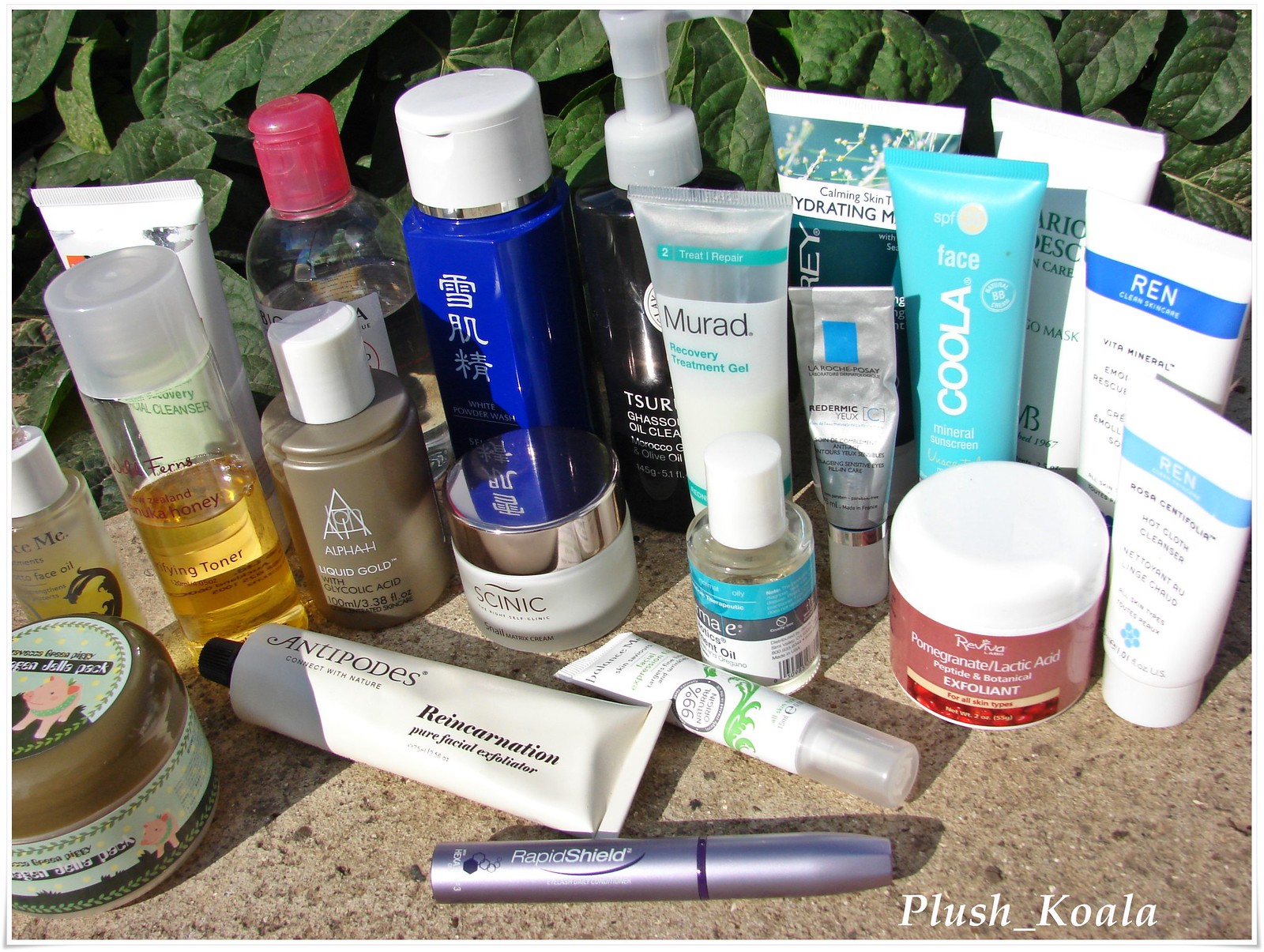This outdoor photograph showcases a diverse collection of lotions and beauty items arranged on a brown and black granite surface. The background features lush green foliage, indicating it was taken outside. In the lower right-hand corner, a watermark reading "Plush Koala" is visible. The assortment includes various brands such as Antipodes, Reincarnation, Rapid Shield, Exfoliant, and Mirad. The products come in different sizes and have an array of colorful labels. Some items appear high-end, while others seem more budget-friendly. Evidence of use is apparent, as one tube is noticeably squished and a bottle is half-empty, suggesting this is a personal collection of beauty products.